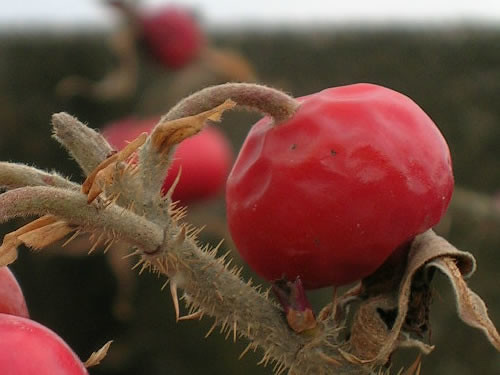In this detailed close-up image, we see a decaying tomato attached to a thorny stem, possibly part of a cactus. The tomato appears squashed and extremely soft, indicating it's near the end of its life cycle and may soon fall off the branch. The stem is covered with numerous small, sharp brown prickles, adding to the overall rugged appearance. The featured tomato, with several pronounced dents—up to nine in total—draws immediate attention due to its deteriorating state. In the background, other tomatoes can be vaguely seen, though they are blurred, highlighting that the focal point is the withering tomato. A glimpse of a healthier red tomato is visible in the lower left corner, contrasting with the browning leaves and stem that encase the central, dying fruit.